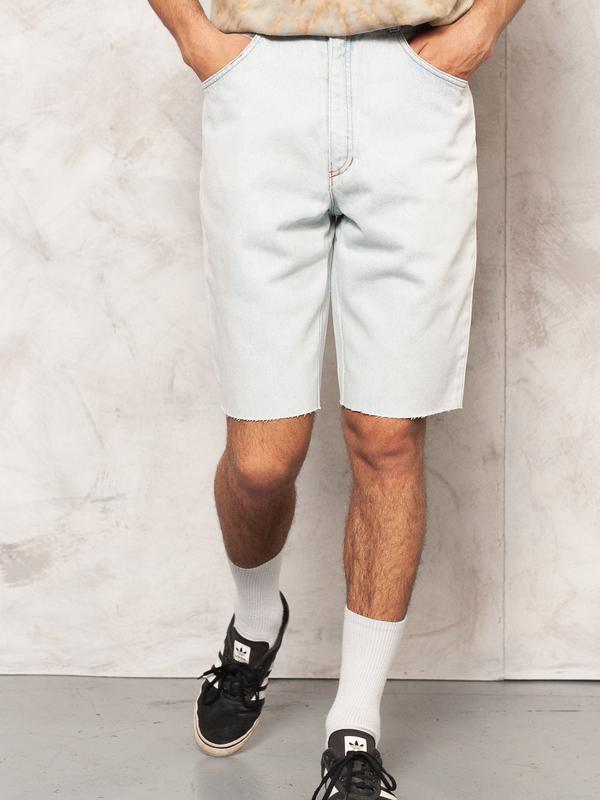This image appears to be an advertisement for clothing, featuring the lower half of a man. He is dressed in a tan, patterned sweatshirt, though only a small part of it is visible. His hands are casually placed in the pockets of his whitewashed jean shorts, which are cut off just above the knee and feature a high-waisted design with a long zipper and prominent seams. His legs, which are semi-hairy and tan, are adorned with high white socks that reach his calves. He is wearing black and white Adidas low-top sneakers. The flooring beneath him is gray, while the background features a marbleized effect in shades of white and gray. The man's stance suggests he is in mid-step, with one foot forward and the other positioned behind, giving the impression of walking forward.